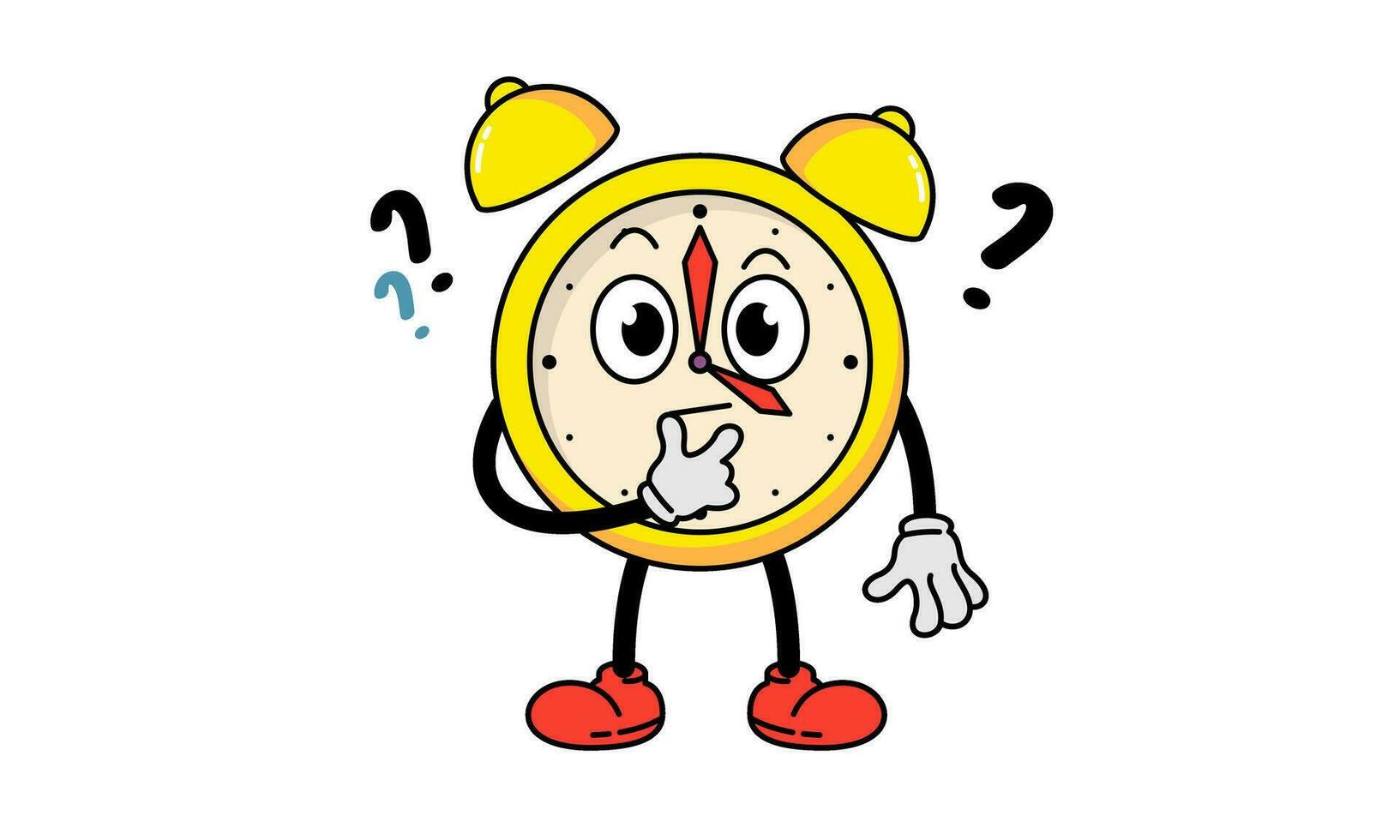The image depicts a cartoon-style drawing of a classic gold alarm clock set against a pure white background. The clock has a circular body, featuring a human-like face with large white eyes, arched eyebrows, and a straight horizontal line for a mouth, giving it a puzzled expression. Extending from the clock are black line arms with white-gloved hands, one of which is touching its face as if rubbing its chin in thought. The clock also has long spindly black legs ending in red shoes. Above the clock face are two traditional alarm bells. Surrounding the clock are three question marks, implying that it is trying to figure something out or is in a state of confusion.